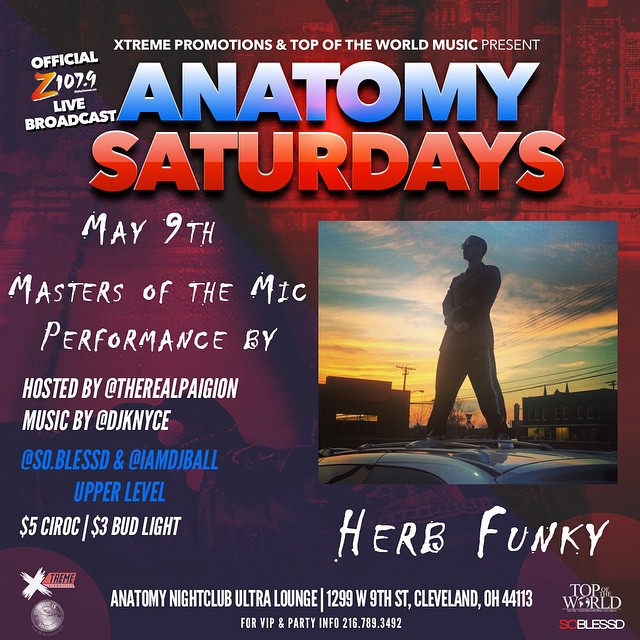This vibrant and eye-catching advertisement, likely from a website or printed on glossy paper, showcases a red and purple-themed poster promoting an event at Anatomy Nightclub Ultra Lounge. At the top, the poster features small white text announcing an official Z107.9 live broadcast brought to you by Extreme Promotions and On Top of the World Music. Dominating the design, the words "Anatomy" in bold blue letters and "Saturdays" in striking red letters highlight the event's name and regular occurrence.

The left side of the poster provides critical event details in white text, stating "May 9th, Masters of the Mic," a performance headlined by Herb Funky. The event is hosted by The Real Pagan and DJ Nice (KNYCE), with additional mentions of social media handles @SoBlessed and @IAmDJBall. Also noted is the special offer of $5 Ciroc and $3 Bud Light. 

On the right side, a central image depicts a man standing atop a vehicle against a sunset backdrop, enhancing the promotional allure. Below this silhouette, the text spells out "Herb Funky" in a distinctive font. The bottom section provides venue information: Anatomy Nightclub Ultra Lounge, located at 1299 West 9th Street, Cleveland, OH 44113, and a contact number for VIP and party information, 216-678-3492.